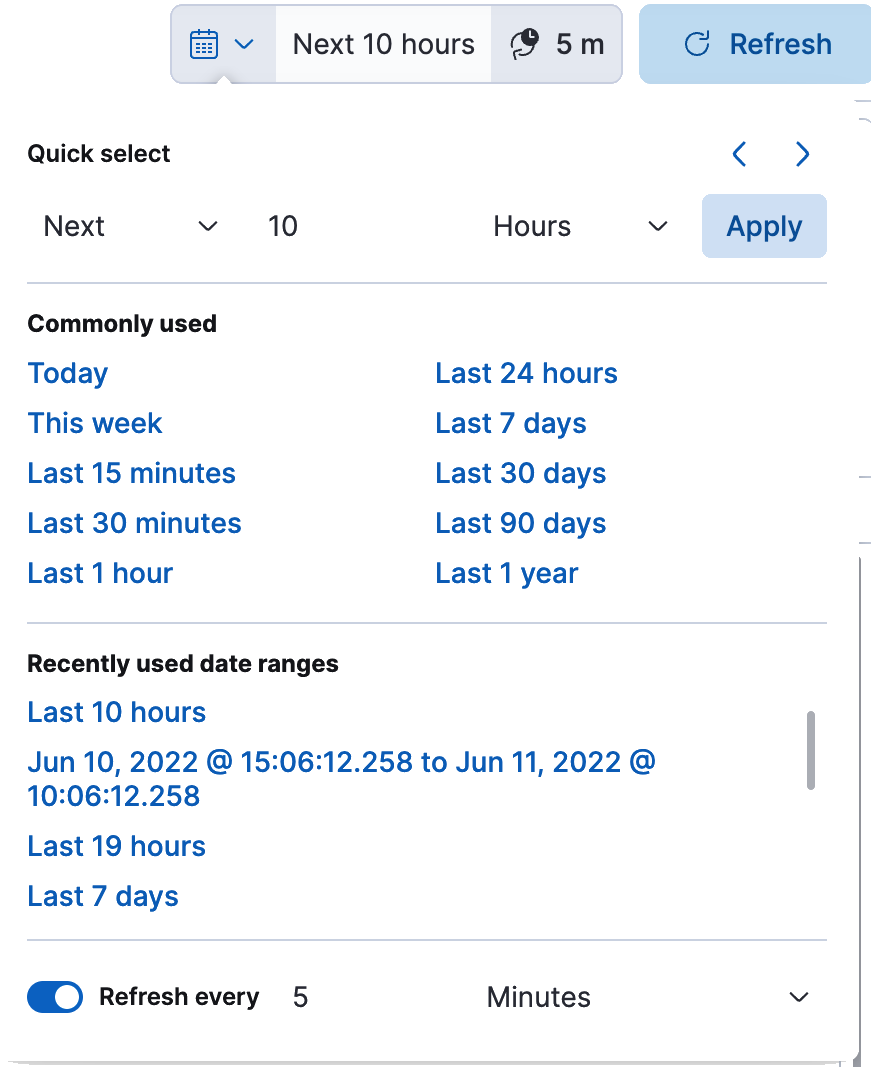The image is a screenshot, likely from a mobile device, though it could also be a cropped section of a website with similar dimensions to a mobile interface. The background is white with predominantly blue text, alongside some black text. At the top left, there's a calendar icon with a drop-down arrow next to it, followed by the text "Next 10 Hours". To its right, there's a blue button featuring a refresh icon and labeled "Refresh". 

Below this, there is a prominently highlighted button in blue with the text "Apply". A section labeled "Commonly Used" is displayed in black text, under which there are several time options listed in blue text: "Today", "This Week", "Last 15 Minutes", "Last 30 Minutes", "Last 1 Hour", "Last 24 Hours", "Last 7 Days", "Last 30 Days", "Last 90 Days", "Last 1 Year".

Further down, a section titled "Recently Used Date Ranges" is shown in black text. This section lists the following options in blue text:

- Last 10 Hours
- June 10, 2022, at 15:06:12.258 to June 11, 2022, at 10:06:12.258
- Last 19 Hours
- Last 7 Days

At the bottom of the screenshot, a toggle switch is shown in blue, indicating it is turned on, with the label "Refresh Every 5 Minutes".